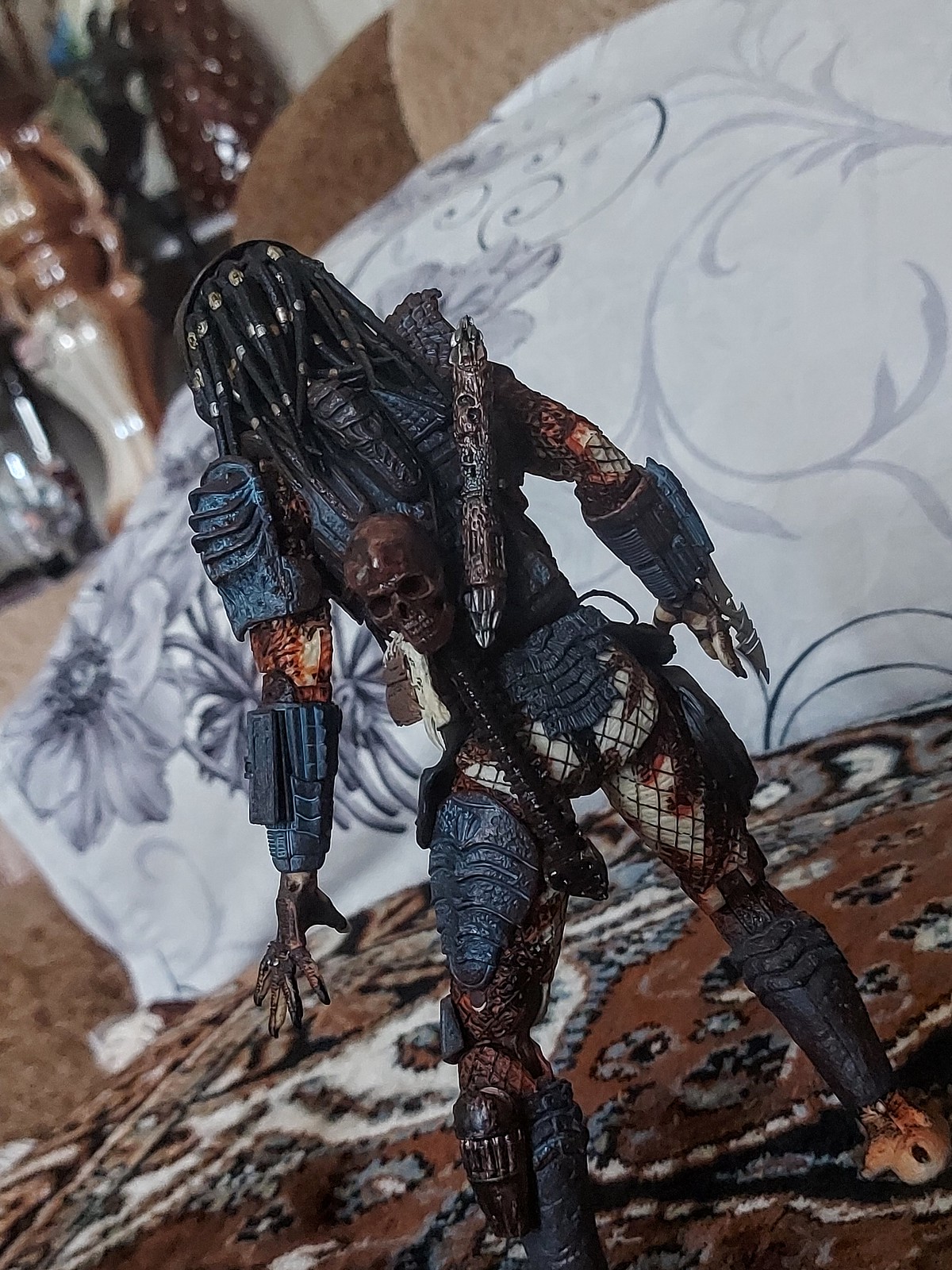This image features a highly detailed action figure of the Predator character from the Predator vs. Alien movies, standing on a multicolored, Persian-style rug. The figure's black braided hair cascades down its back as it faces away from the viewer. The composition is slightly tilted to the left, with the head towards the top left and the legs angled towards the bottom right. Reinforcing its menacing appearance, the Predator wears intricate blue and black armor, with additional straps of mesh-like material overlaying red and white, fish-like skin. Distinctive weaponry is attached to its forearms: sharp claws on the right and a mysterious device on the left. On its back, there's both an image of a skull and what appears to be another weapon. The scene's background includes a white pillow, a bedpost, and some carpet, adding depth to the setting.